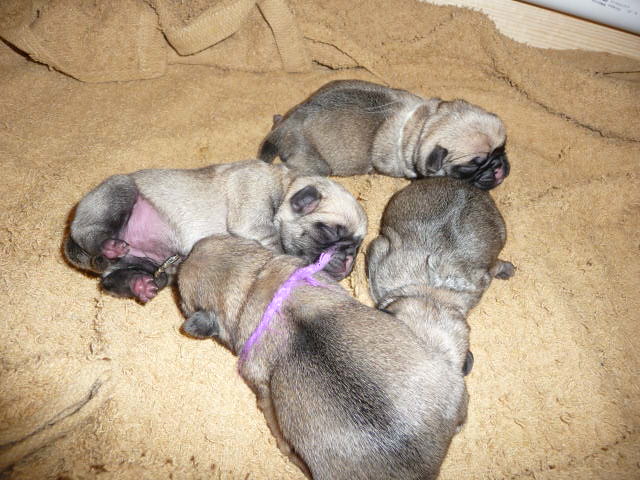This image features four newborn puppies, likely pugs, all peacefully asleep. They are lying on a soft, beige towel that rests on a pale hardwood floor. Each puppy has a small pink or purple neck band, adding a touch of color to their mostly brindle (brown and beige) fur. The puppies have tiny, round, dark ears and darker masks around their muzzles and eyes. One puppy is lying on its side, exposing its little pink belly and the undersides of its pink feet. The scene is heartwarmingly cute, with all four puppies nestled close together on the towel.